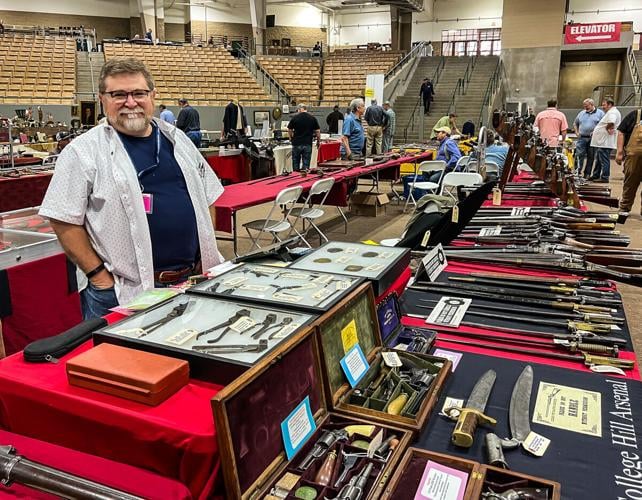In this detailed indoor color photograph, a man stands smiling in the foreground of a trade show set in a gymnasium, evident from the bleachers with brown seats rising in layers behind him. He sports sandy-colored hair, glasses, a short goatee, and is dressed in a navy blue t-shirt beneath an unbuttoned white collared short-sleeve shirt. He completes his look with denim pants and a brown belt, his hands resting casually in his pockets. The gym floor is arranged with numerous tables draped in red tablecloths, each displaying an array of historical artifacts, including swords, knives, bayonets, muskets, and pistols. Some items are housed in cases, while others lie directly on the table coverings. Text on one of the tables reads "College Hill Arsenal," suggesting a focus on historical weaponry. Surrounding the man, one can see white folding chairs and more attendees examining the exhibits, contributing to the bustling yet scholarly atmosphere of the convention.